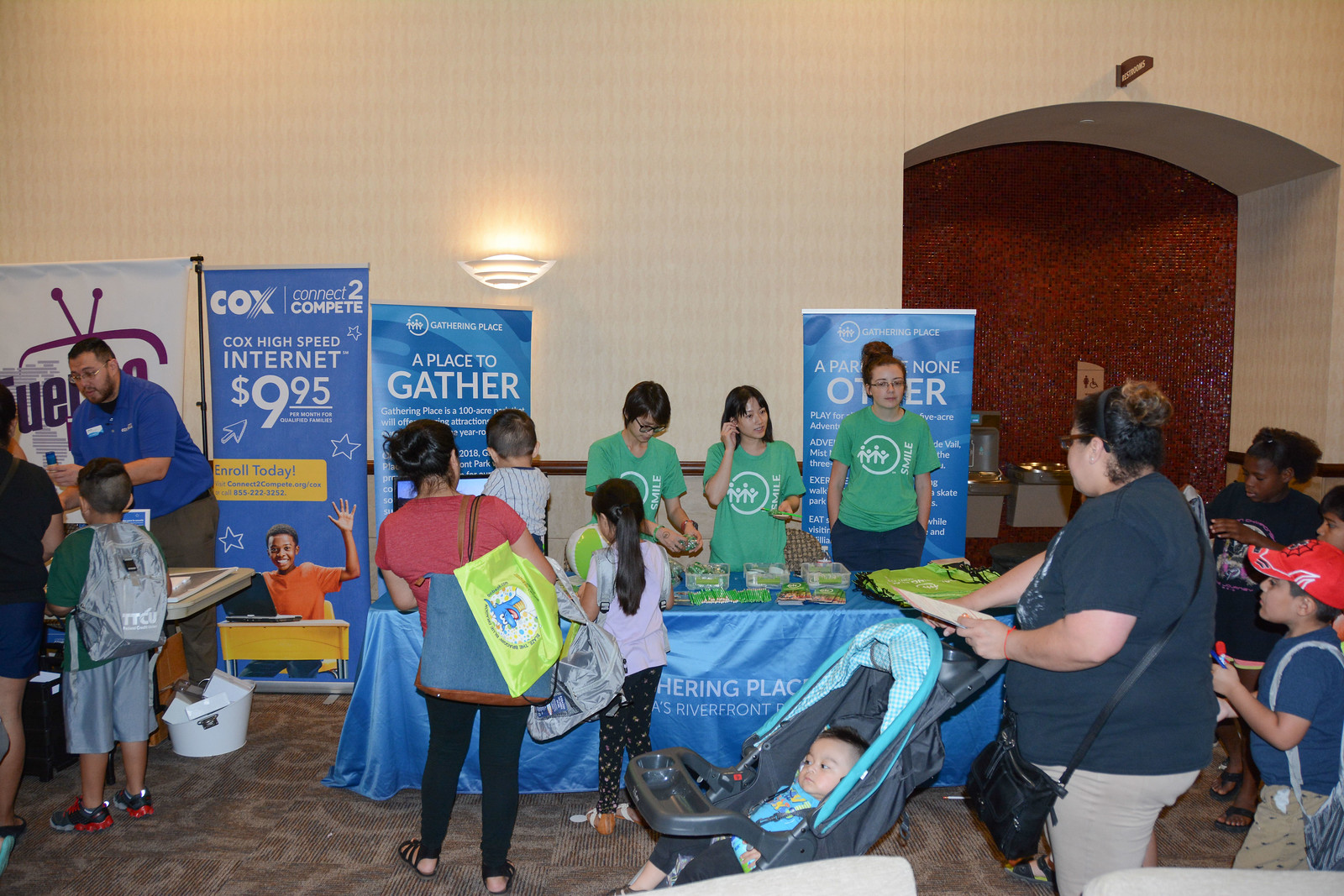In this detailed indoor scene set within a convention center or school hall, we see a bustling, vibrant environment captured in a wide rectangular photograph. Central to the image is a table draped in a shiny blue tablecloth, behind which stand three young women, likely in their early teens, and an older woman who could be a teacher or mentor, all wearing green t-shirts with a white circular logo. The women are engaged in what seems to be a community or educational event.

In front of their table, a young child around eight years old, with her back to the camera, appears captivated by the display. Nearby is a woman in an orange shirt holding a baby and carrying a large tote bag. She is followed by another woman with a black purse, pushing a baby in a stroller, and a child wearing a red baseball cap.

To the left of the green-shirted group, several prominent signs catch the eye. One reads "Cox Internet 995" and another says "A Place to Gather, Gathering Place." Adjacent to these signs is another table manned by a man in a blue shirt, with a TV antenna banner behind him. A child with gray shorts and a backpack looks on, interested in the man's display. The backdrop of the image includes a door, a white wall adorned with a sconce, and an indent in the wall with a dark reddish-brown background. The carpeting visible at the bottom left corner is brown with light brown shading, adding a subtle texture to the indoor environment.